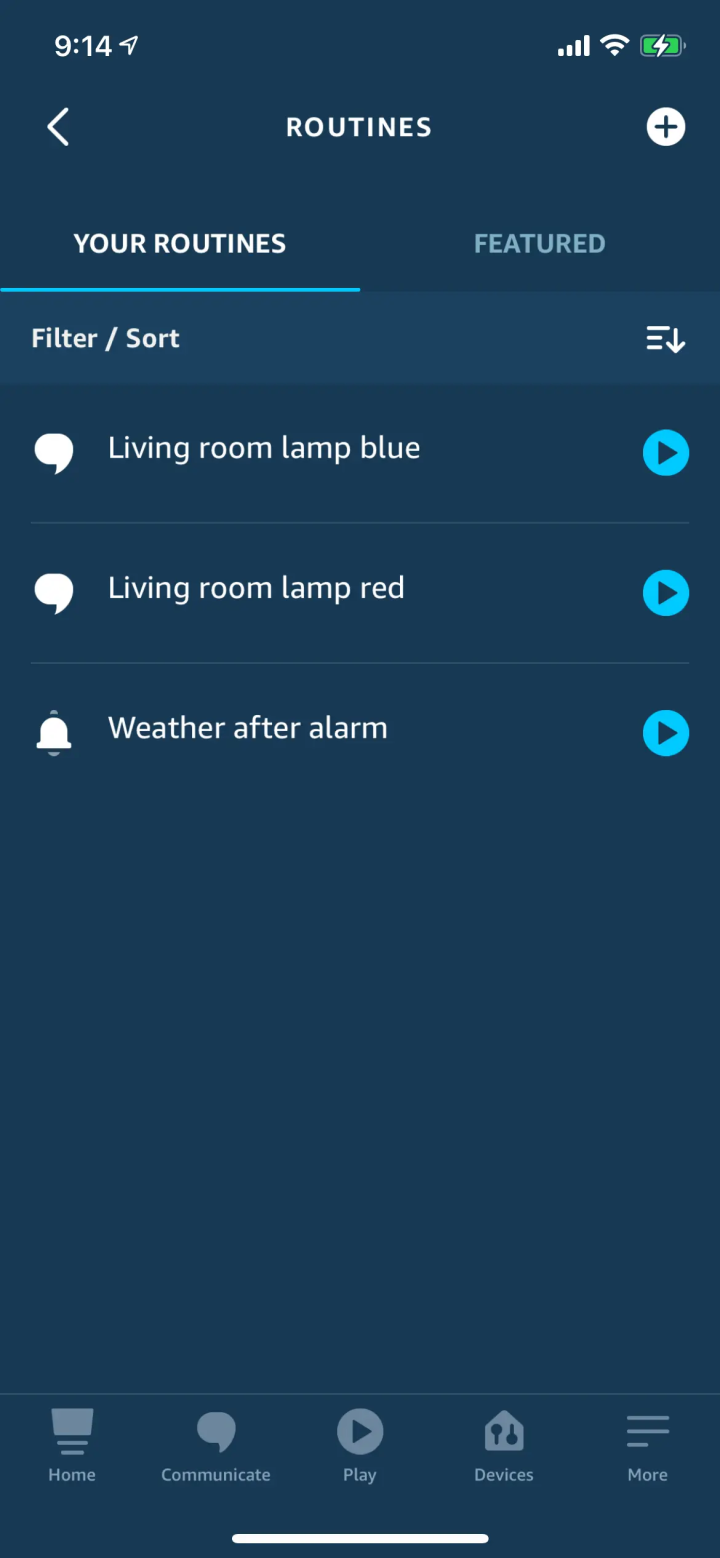This image is a full-color screenshot of a smartphone displaying an app interface. The time shown is 9:14 AM, indicated at the top of the screen along with icons for full cellular reception, Wi-Fi, and a fully charged battery, symbolized by a green icon. The app in view appears to be one for managing routines, evidenced by the "Routines" label at the top. 

The user has two tabs to choose from: "Your Routines" and "Featured," with sorting options available. Three routines are listed in the screenshot: "Living Room Lamp - Blue," "Living Room Lamp - Red," and "Weather After Alarm." Each routine features a play button next to it, presented as a light blue circle with a dark blue arrow in the center. 

The app's background is a navy blue with white text, creating a high-contrast and easily readable display. At the bottom of the screen, there are navigation icons allowing the user to switch between "Home," "Communicate," "Play," "Devices," and "More," facilitating easy access to different sections of the app.